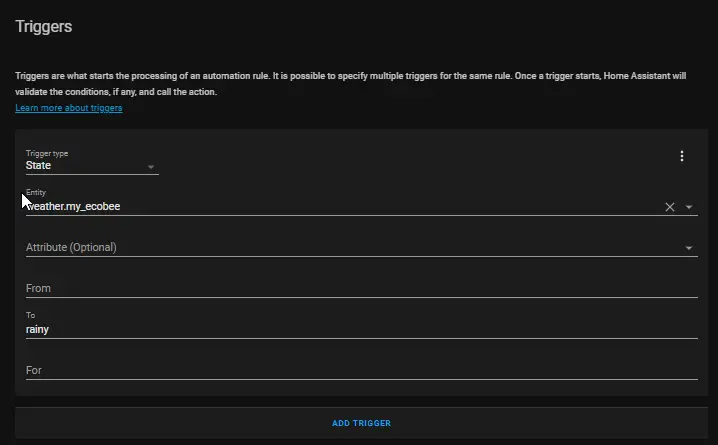A black screen with a minimalistic interface is displayed, providing a clean and user-friendly experience. In the upper left-hand corner, the word "Triggers" is highlighted in a gray font with a capital 'T'. Below, an informational paragraph explains the function of triggers in Home Assistant, detailing how triggers initiate the automation rule process. It reads: 

"Triggers are what starts the process of an automation rule. It is possible to specify multiple triggers for the same rule. Once a trigger starts, Home Assistant will validate the conditions, if any, and call the action."

A clickable link in blue text, "Learn More About Triggers," offers additional information for those who wish to delve deeper.

Moving down, the first form field labeled "Trigger Type" shows a drop-down menu with the default option "State" selected. Next to "Trigger Type," an icon featuring three dots allows access to more details.

The following line includes the "Entity" field set to "Weather.My.EchoV," with options to clear or select from a drop-down menu. The optional "Attribute" field also provides a drop-down menu for user selection.

Further down, fields labeled "From" and "To" are present. The "From" field is empty, while the "To" field is populated with the word "Rainy." The last field, "For," is currently empty.

At the bottom, centre-aligned in blue capital letters, the button "ADD TRIGGER" invites users to finalize their trigger setup.